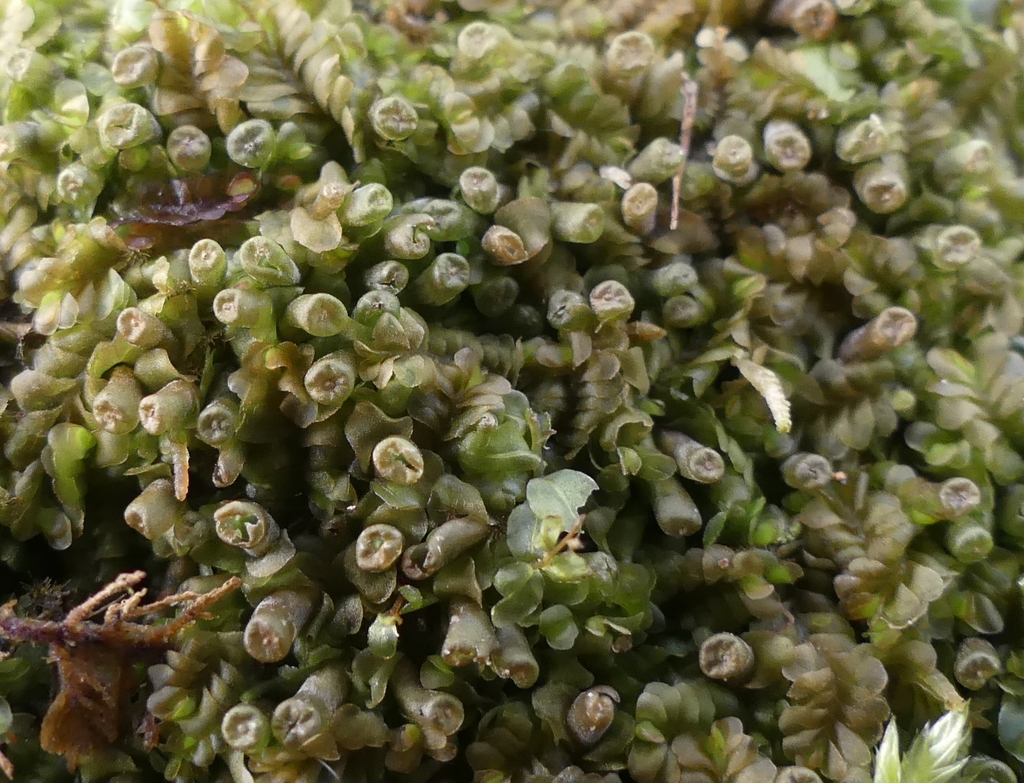This detailed close-up image showcases a dense, intricate structure resembling the severed ends of various green plant stems, arranged in a somewhat spherical formation, though not fully visible. The plant appears to grow in water, indicated by its green, brown, and beige hues. The ends of these stems are puckered and ragged, reminiscent of dried or sliced jalapenos, green onions, or perhaps even frozen green or white grapes. The arrangement of the plant parts gives them a rolled, almost tornado-like appearance. In the bottom left corner, there is a prominent twig-like structure, while from the lower right corner, various leaves extend upward. A similar brownish foliage can be observed in the top left corner, contributing to the overall textured and layered composition of the image.